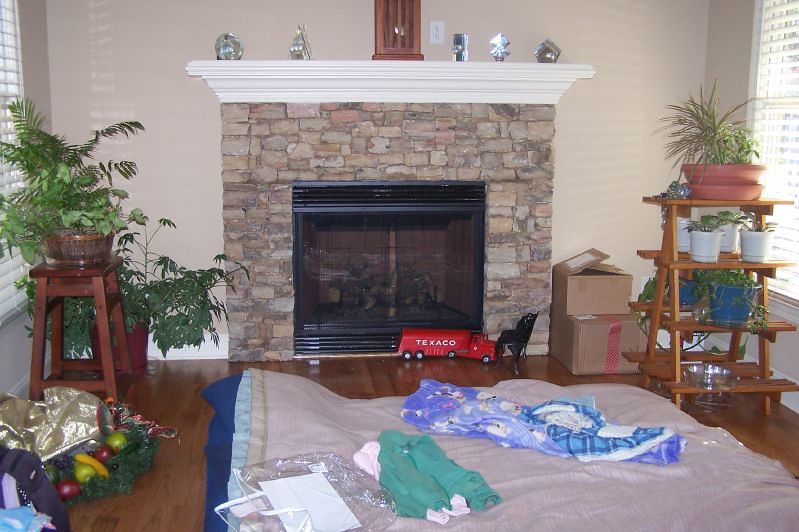This image depicts a living room, which appears to be in a state of transition, possibly due to moving in or packing up. The focal point is a fireplace with a stone brick facade and a white mantle adorned with various shiny awards or trinkets. The fireplace itself shows signs of previous use with blackened logs and a black front grid. To the left of the fireplace, there are two potted plants, one placed on a stand and the other on the ground; both are green and leafy. In front of the fireplace, a red Texaco toy truck and a small black chair, possibly a kid's toy, are visible. 

To the right of the fireplace, there are two cardboard boxes, one open and the other taped shut. Beyond these boxes, a multi-tiered wooden stand holds more potted plants. These plants are in pots of various colors: pink, white, blue, with vines, and a built-in watering system at the bottom. A matching planter setup is also present on the left side of the room, backed by a window. 

An air mattress, colored blue, occupies the center of the room, draped with a blue and pink blanket. Nearby, there is a jacket that is green and white and another blanket in blue and white, rolled up. Additionally, on the right side of the image, a wreath decorated with fake fruit adds a unique element to the scene.